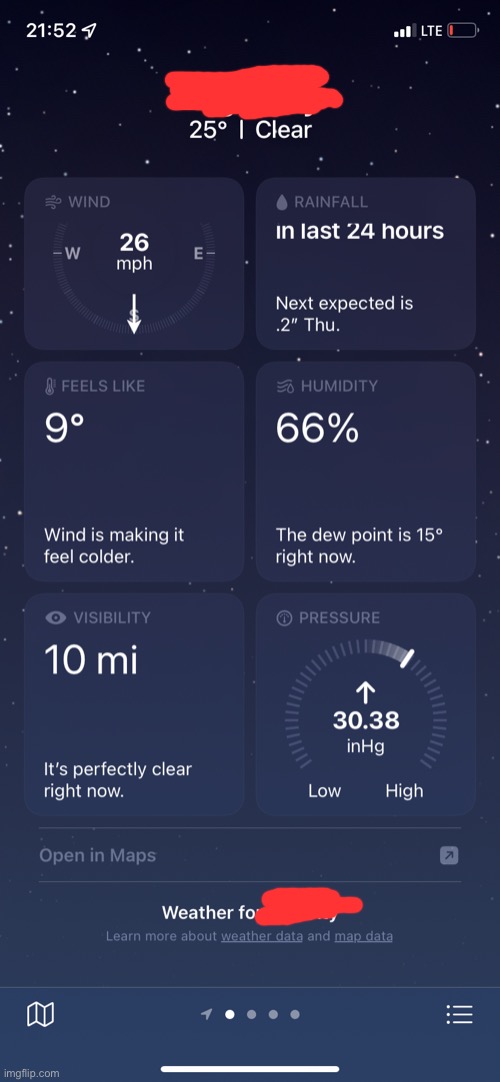This image is a detailed screenshot from a cellphone, showcasing a weather app at night. 

The background simulates a night sky adorned with numerous stars of varying sizes, predominantly in shades of blue and white. At the top of the screen, the status bar displays the time as 21:52 along with icons indicating a strong cellular signal, LTE connectivity, and a battery level that is low, featuring a small red segment. The location name has been digitally obscured with a red marker.

Below the status bar, the temperature is indicated as 25 degrees. A horizontal line runs across the center of the screen with the word "clear" positioned on the right side, suggesting clear weather conditions.

Structured into two columns of three, the screen includes several informative widgets:
- The top left widget indicates the wind speed as 26 miles per hour coming from the south.
- Adjacent to that, on the right, it notes the recent rainfall with a next expected amount of 0.2 inches on Thursday.

The second row continues with:
- The left widget stating it "feels like 9 degrees" due to the wind chill factor.
- On the right, the humidity level is given as 66%, with a dew point of 15 degrees.

The final row informs:
- The left widget provides visibility at 10 miles, describing the current conditions as perfectly clear.
- The right widget details the atmospheric pressure as 30.38 inches of mercury (IN8HG), presenting it on a scale from low to high.

At the bottom of the screen, there is a prompt to "open in maps" and a partially obscured label indicating the weather information source, labeled as "Weather 4."